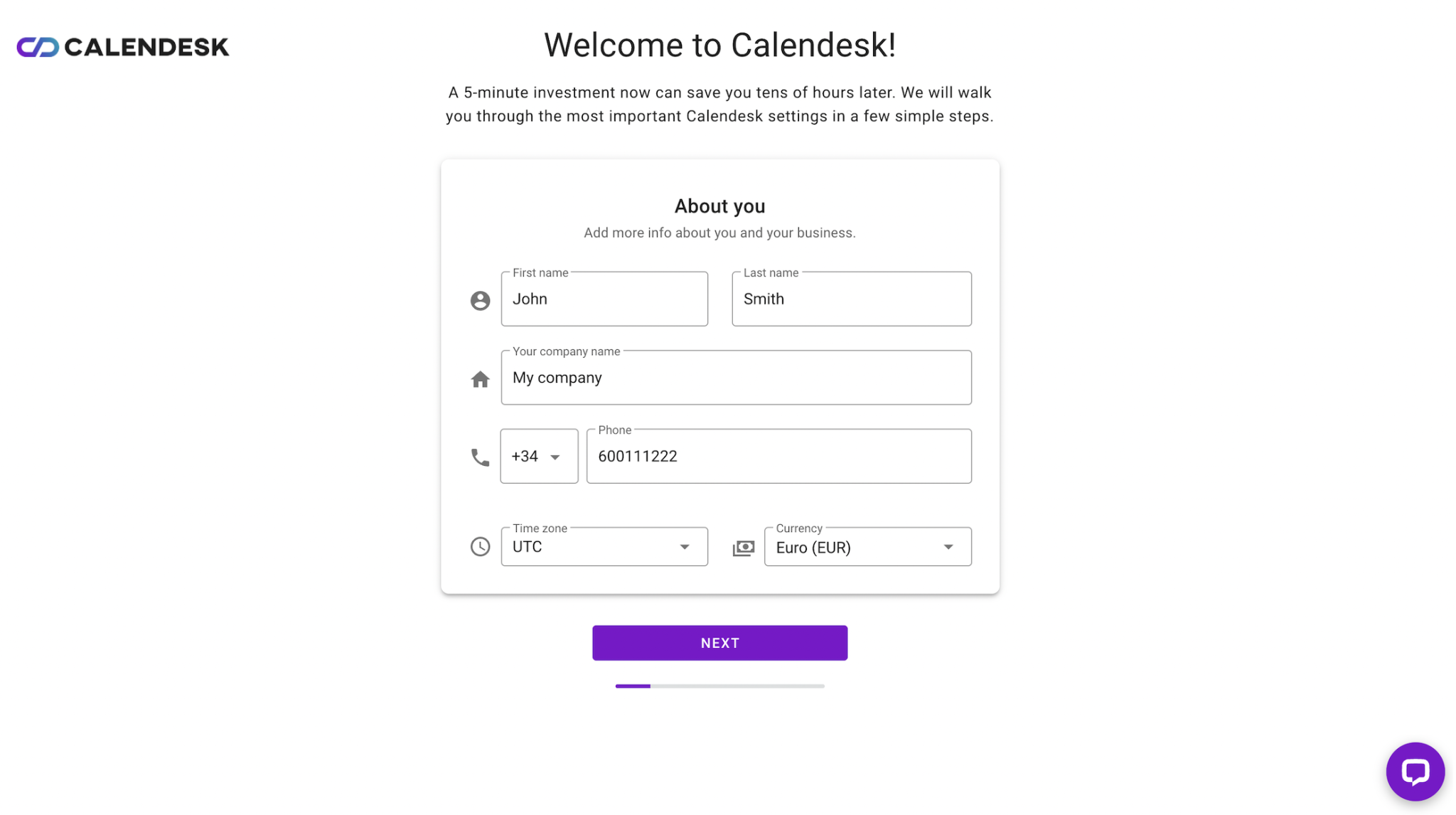This screenshot depicts a webpage from the Calendesk platform, primarily dominated by a clean, white interface enhanced by minimalistic design elements. In the top left corner, a logo featuring a stylized infinity symbol (resembling a sideways 'S') in purple and teal hues is prominently displayed, accompanied by the word "Calendesk" in bold black letters. 

Centrally positioned on the page is a welcoming message: "Welcome to Calendesk!" followed by the text, "A five-minute investment now can save you tens of hours later. We will walk you through the most important Calendesk settings in a few simple steps." Below this message is a section enclosed within a square titled "About you," prompting users to provide personal and business information. Fields for first name, last name, company name, a field marked as "+34" (presumably for an age or phone prefix), phone number, time zone, and preferred currency (defaulting to "Euro," indicated alongside dollar signs) are present.

At the bottom of this section, there is a prominent "Next" button in purple. Additionally, a horizontal progress indicator is displayed, with a gray line partially filled with purple on the left end. In the bottom right corner, a purple speech bubble icon likely indicates a chat or help feature.